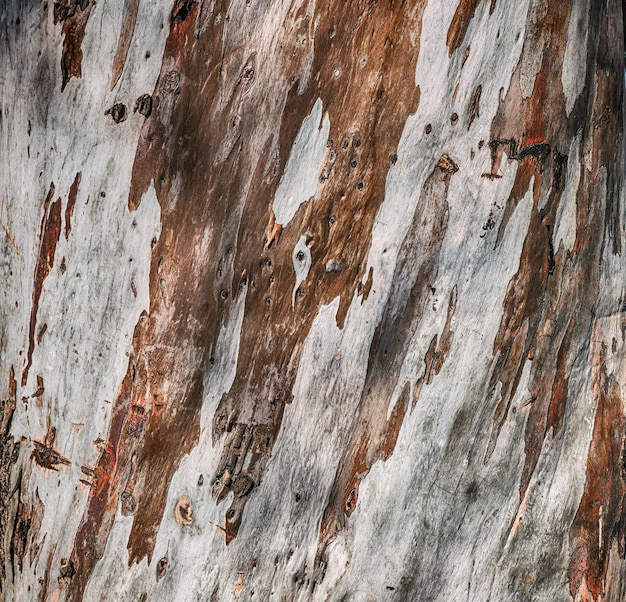The image is a close-up photograph of tree bark featuring a predominantly brown surface with intricate, irregular white streaks running through it, giving the impression that they were painted on. The two contrasting colors create a visually striking pattern, where the white streaks are vertical and slightly slanted. Adding to the complexity, the bark displays various wormholes and carvings, indicating possible damage from insects or other elements. Despite the rough appearance and tactile textures suggested by the markings, part of the bark exhibits a smoother surface. There are also dark brown spots and areas where the grayish bark seems chipped away, contributing to the rich detail and dynamic nature of the photograph.